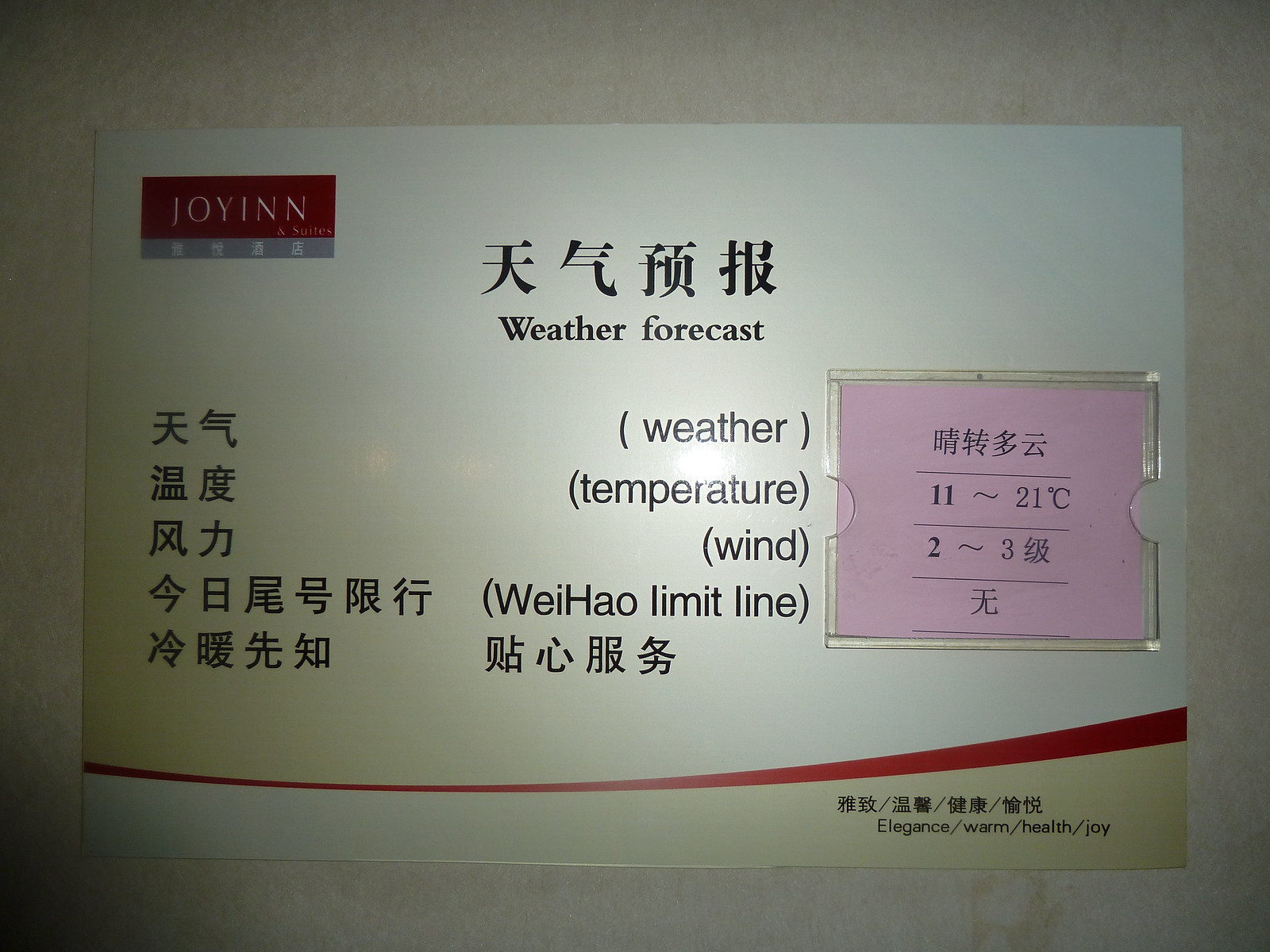The image depicts a sign mounted on a speckled grey and dark grey wall, likely in a hotel setting. The sign is primarily grey, featuring a gradient effect from the top right to the bottom left corner and is divided into two sections, with the lower one-fifth having a curved red line. In the top left corner, a red rectangular logo reads "JOYINN & SUITES." At the top center of the sign, large text in both Chinese and English declares, "Weather Forecast." The rest of the sign is organized into sections labeled "Weather," "Temperature," "Wind," and "Weihao Limit Line," with all headings replicated in both Japanese and English. The temperature is listed as ranging from 11 to 21 degrees Celsius, and the wind as 2 to 3. Along the bottom right-hand corner of the sign are Chinese words that translate to "Elegance," "Warm," "Health," and "Joy." The detailed presentation highlights information likely intended for guests, providing weather details in a clear, bilingual format.